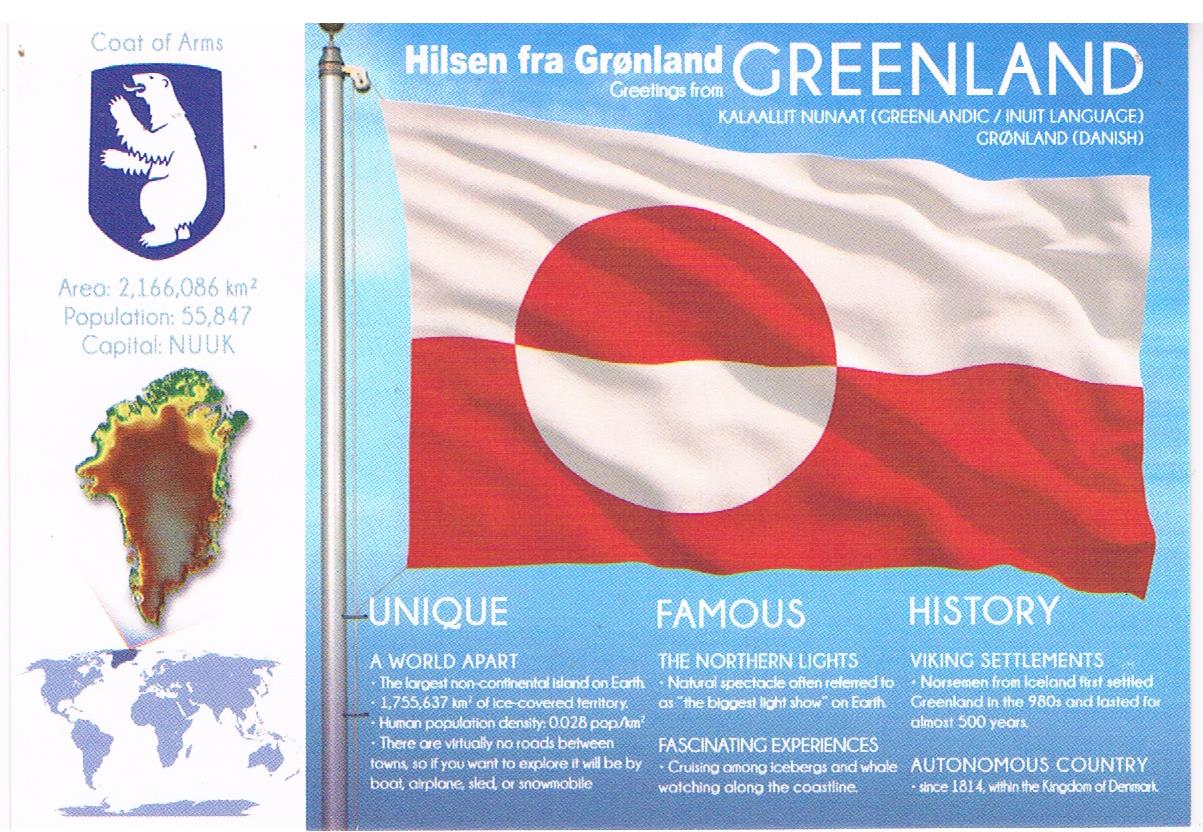This infographic provides a comprehensive overview of Greenland, blending text, images, and graphics into a cohesive layout. The left quarter of the image is a vertical white section featuring Greenland's coat of arms on a blue background with a white polar bear, accompanied by textual details including its area (2,166,086 km²), population (55,847), and the capital city, Nuuk. Beneath these statistics, there's a heat-mapped close-up of Greenland and a world map highlighting its location.

The remaining right portion of the graphic, set against a blue backdrop, prominently displays Greenland's flag. The flag is characterized by a white horizontal stripe at the top, a red stripe at the bottom, and a unique circle on the left third with inverted colors—white on the red portion and red on the white portion. In white text, the word "Greenland" is displayed along with possibly its name in Inuit language and Danish.

At the bottom of the infographic, three columns labeled "Unique," "Famous," and "History" outline key aspects of Greenland. These include its Northern Lights, Viking settlements, and its status as an autonomous country. This section underscores Greenland's distinctive features, historical significance, and notable attractions, making the infographic an informative promotional material for Greenland.